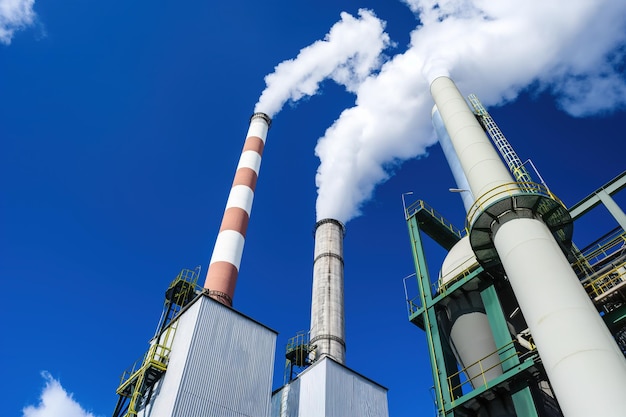The image depicts a low-angle shot, capturing the towering structures of a power plant or industrial refinery. Dominating the frame are four smokestacks of varying heights and appearances, each emitting bright white steam against a vivid blue sky. The most striking of these is decorated with red and white bands, while the others are primarily concrete, with two appearing darker in color. Surrounding the smokestacks are interconnected industrial elements, including a nearby white silo adorned with a green trellis of stairs and walkways, designed for workers' access. The base of the smokestacks features buildings equipped with ladders and stairs, further emphasizing the complex and functional nature of this facility. The contrast between the industrial machinery and the clear sky adds a unique aesthetic quality to the scene.